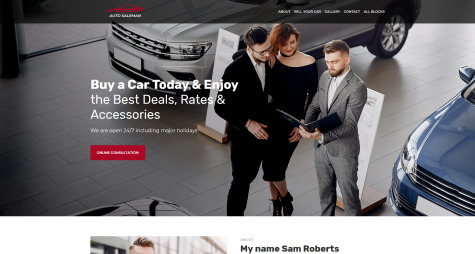A screenshot from a car sales website captures the scene inside a dealership showroom. At the top of the page, a partially obscured red car logo is visible, immediately followed by a semi-transparent gray menu on the right. Dominating the upper portion of the image, a primary photograph shows a man and a woman in conversation with a professional car salesman. The salesman is holding and pointing to a black book, presumably containing the car's specifications and details. Surrounding them, several cars are on display within the modern and well-lit showroom.

To the left of the image, bold white text reads, "Buy a car today and enjoy the best deals, rates, and accessories," accompanied by a smaller, illegible block of text beneath it. Below the promotional message is a prominent red button, also bearing some unreadable text.

Further down, the layout transitions into a new section, beginning with the introductory sentence, "My name is Sam Roberts," though no additional context follows. A partially cropped photograph, likely of Sam Roberts, is included but not fully visible, leaving some speculation about his identity and role in the dealership.